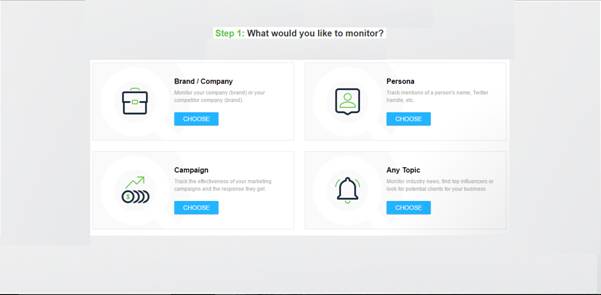This image features a light gray, horizontally elongated rectangle with a thin black line at the very bottom. Centered at the top, the text "Step One: What would you like to monitor?" is prominently displayed in green and black. Within the main area of the image, four smaller rectangles are arranged in a 2x2 grid.

1. **Top Left Rectangle:**
   - Contains the label "Brand/Company."
   - Features an icon resembling a briefcase.
   - Includes some text that is not fully readable and a blue button likely labeled "Choose."

2. **Top Right Rectangle:**
   - Labeled "Persona" with a person icon adjacent to it.
   - Some unreadable text present along with a similar blue "Choose" button.

3. **Bottom Left Rectangle:**
   - Titled "Campaign" and includes an icon of money with a green upward arrow.
   - Contains illegible text and a blue button that mirrors the "Choose" label.

4. **Bottom Right Rectangle:**
   - Features the label "Any Topic" accompanied by a bell notification icon.
   - Contains some unreadable text and a blue button, presumably also labeled "Choose."

There are no additional indications of the image’s context, medium (whether it’s from a cell phone, tablet, or computer), or specific application.